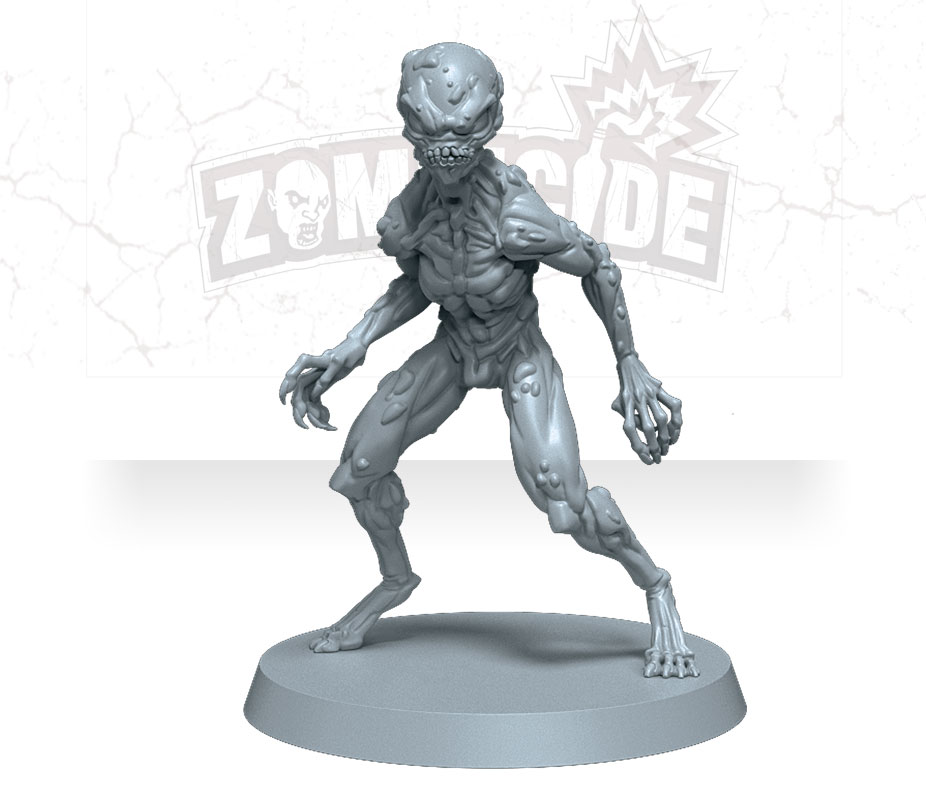This image features a highly detailed, gray 3D-printed model replica of a fictional alien or zombie character. The figurine showcases an intricate design, with exposed muscular structures on its shoulders, chest, legs, toes, and fingers, resembling an alien with large, menacing teeth, and alien eyes. Its head is adorned with rounded baubles and numerous bumps, adding to its ferocious appearance. Standing on a round, matte gray platform, the character strikes a formidable stance. In the background, on a white surface, there is a faint watermark displaying the logo for "Zombicide" in black and white. The O in "Zombicide" is depicted as a zombie face, and the I in "side" resembles a lit Molotov cocktail or dynamite stick. The backdrop also features subtle wall cracks, completing the eerie and ominous scene.